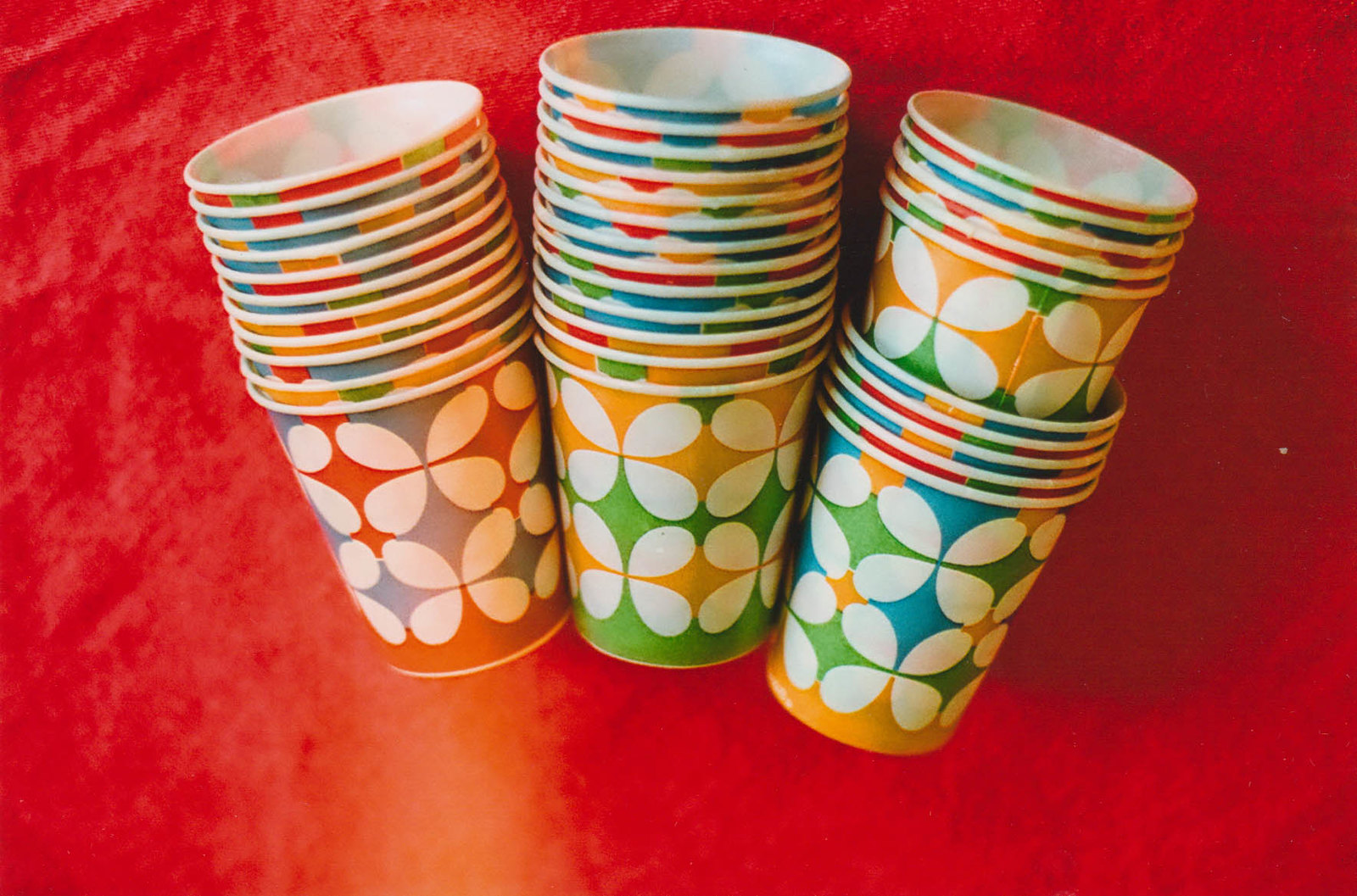The image features a close-up view of three horizontally aligned stacks of paper cups, vividly set against a rich red background that resembles a tablecloth or a fabric draped over a surface. The stacks, decreasing in size from left to right, each contain roughly 10 to 15 cups and lie on their sides rather than standing upright. The cups are brightly colored and decorated with a cheerful, intricate design that evokes feelings of picnics and parties. The design consists of a four-pronged star shape overlaid on a circular pattern, creating a series of white petal-like shapes that encircle the cups in two neat rows—one at the top and one at the bottom. The background's appealing red hue is complemented by subtle touches of yellow and pale yellow, while the cups themselves feature a multicolor palette with shades of red, orange, green, blue, and some white within the floral patterns. Despite the photograph not being of super high definition, the details of the vibrant and festive imagery are clearly discernible, with no text marring the aesthetic appeal of the scene.